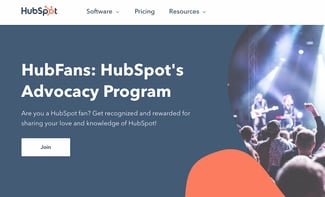The image is a small, horizontal rectangle with a distinct structure. The uppermost section features a white horizontal rectangular area, which serves as the background for the website's header. Prominently positioned is the name "HubSpot" with "Hub" and "Spot" in black and the "O" in orange. To the right of the site name are three menu items labeled "Software," "Pricing," and "Resources," each accompanied by a small arrow suggesting a dropdown menu.

Below this, the main section of the image has a blue background with bold white text that reads, "HubFans: HubSpot's Advocacy Program." In smaller white font beneath, a tagline invites users to become part of the community: "Are you a HubSpot fan? Get recognized and rewarded for sharing your love and knowledge of HubSpot." 

Positioned further down is a small white rectangle that bears the word "Join" in black text, centered within it. To the right side of the main blue area, an image extends down in a semi-circular shape. This image captures a vibrant concert scene, with a performer playing the guitar on stage illuminated by bright lights, creating a visual glare. The backs of the audience members are visible, with one arm raised in the air, emphasizing the energy of the event.

The bottom left corner of the image features a plain orange element, resembling the shape of a thumbprint, though it is cut off at the bottom, adding a splash of color and texture to the design.